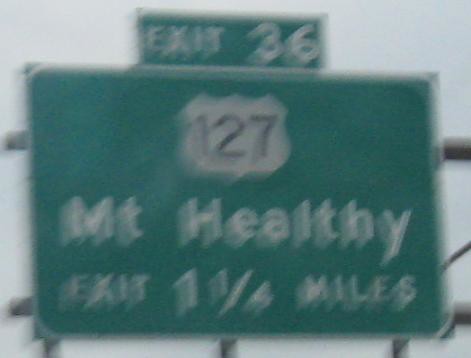Photographed from a moving vehicle, this image shows a blurred highway sign supported by a latticework structure, giving a hazy, out-of-focus appearance due to either camera shake or the vehicle's speed. The green sign indicates an upcoming exit, Exit 36, leading to Mount Healthy, spelled as "M-T-H-E-A-L-T-H-Y", 1.25 miles ahead. It clarifies that this exit connects to Highway 127. The backdrop features an overcast sky, hinting at a possibly busy highway environment.